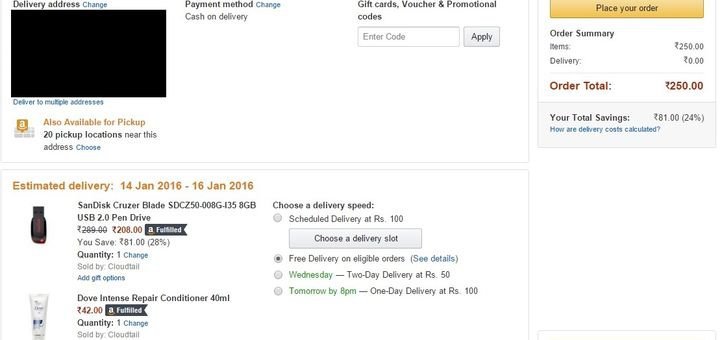**Detailed Caption:**

The screenshot features a user interface with a white background. Key options are highlighted in blue text, including "Delivery address changes," and "Payment method change." Additionally, it indicates options for "Cash on Delivery" and the availability of gift cards, vouchers, and promotional codes. A gray rectangle contains a box labeled "Enter code" with an "Apply" button for entering promotional details.

The interface notes that the order can be delivered to multiple addresses and offers pickup options with 20 available locations near the specified address. There's a blue "Choose" link for selecting a pickup location.

On the right side, a prominent box contains the "Place your order" button in black text within a yellow rectangle. Below this, an order summary is presented:
- Item cost: ₱250
- Delivery cost: ₱0
- Order total: ₱250 (with the second instance of 250 in red)
- Notable savings: ₱81 (24% savings noted in parentheses)

A question mark link asks, "How are delivery costs calculated?" The estimated delivery window is specified as January 14, 2016, to January 16, 2016. At the bottom of the interface, it states, “Sand this cruiser blade.”